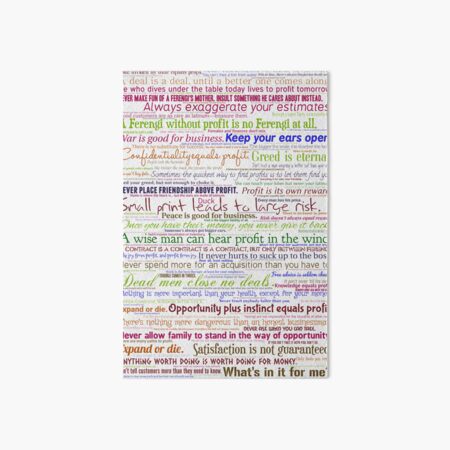The image features a vibrant and eclectic sign or poster set against a white background, filled with an array of colorful and varied text, presenting numerous business-related sayings and "Ferengi Rules to Live By." The text is in multiple colors, including green, pink, blue, orange, brown, and purple. It showcases various fonts and styles, adding to the visual interest. Some of the prominent rules include: "Opportunity plus instinct equals profit," "Satisfaction is not guaranteed," "Expand or die," "What's in it for me?" "Greed is eternal," "A wise man can hear profit in the wind," and "Small print leads to large risk." Other notables are "Always exaggerate your estimates," "War is good for business," and "Never place friendship above profit." There are also Ferengi-centric aphorisms like "A Ferengi without profit is no Ferengi at all," and "Never make fun of a Ferengi's mother, insult something he cares about instead." Some text is slightly blurred or cut off, but the messages emphasize a mercantile philosophy, underscored by the visual variety and the meticulous detail in the presentation.